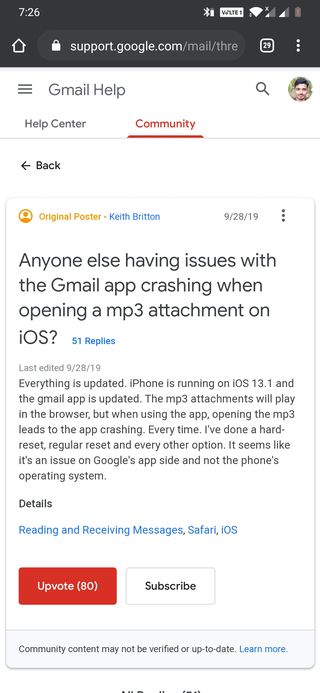This detailed description accompanies a cell phone screenshot of an online forum page, specifically the Gmail Help Community on support.google.com. 

At the very top, a black rectangular bar displays standard smartphone icons, including battery life, time, Wi-Fi, and signal strength indicators. Beneath it, in the upper left corner, there is a white house icon representing the home function next to a search bar. The search bar, showing a white lock icon and the URL "support.google.com/mail/three" in white and gray text, indicates secure browsing.

The main content area has a white background. In the upper left corner, three horizontal gray lines represent the menu icon, while to the right, the title "Gmail Help" is in gray text. On the right side of this header, there are a profile icon and a magnifying glass for search functionality.

Below the header, two options are displayed: "Help Center" and "Community". The "Community" option is highlighted and underlined in red, indicating the current selection.

Further below, a left-pointing arrow followed by the bold black word "Back" allows users to navigate to the previous page. Positioned beneath this, a light gray-outlined rectangle contains a question in gray text: "Anyone else having issues with the Gmail app crashing when opening an MP3 attachment on iOS?"

Following this question, a user's reply in gray text reads: "Everything is updated. iPhone is running on iOS 13.1 and the Gmail app is updated. The MP3 attachments will play in the browser, but when using the app, opening the MP3 leads to the app crashing every time. I've done a hard-reset, regular reset, and every other option. Seems like it's an issue on Google's app side and not on the phone's operating system."

At the bottom of the screen, two rectangular buttons are displayed. The left button is red and contains the text "Update (80)" in white, while the right button is white with "Subscribe" in black text at the center. This indicates user engagement options for the forum post.